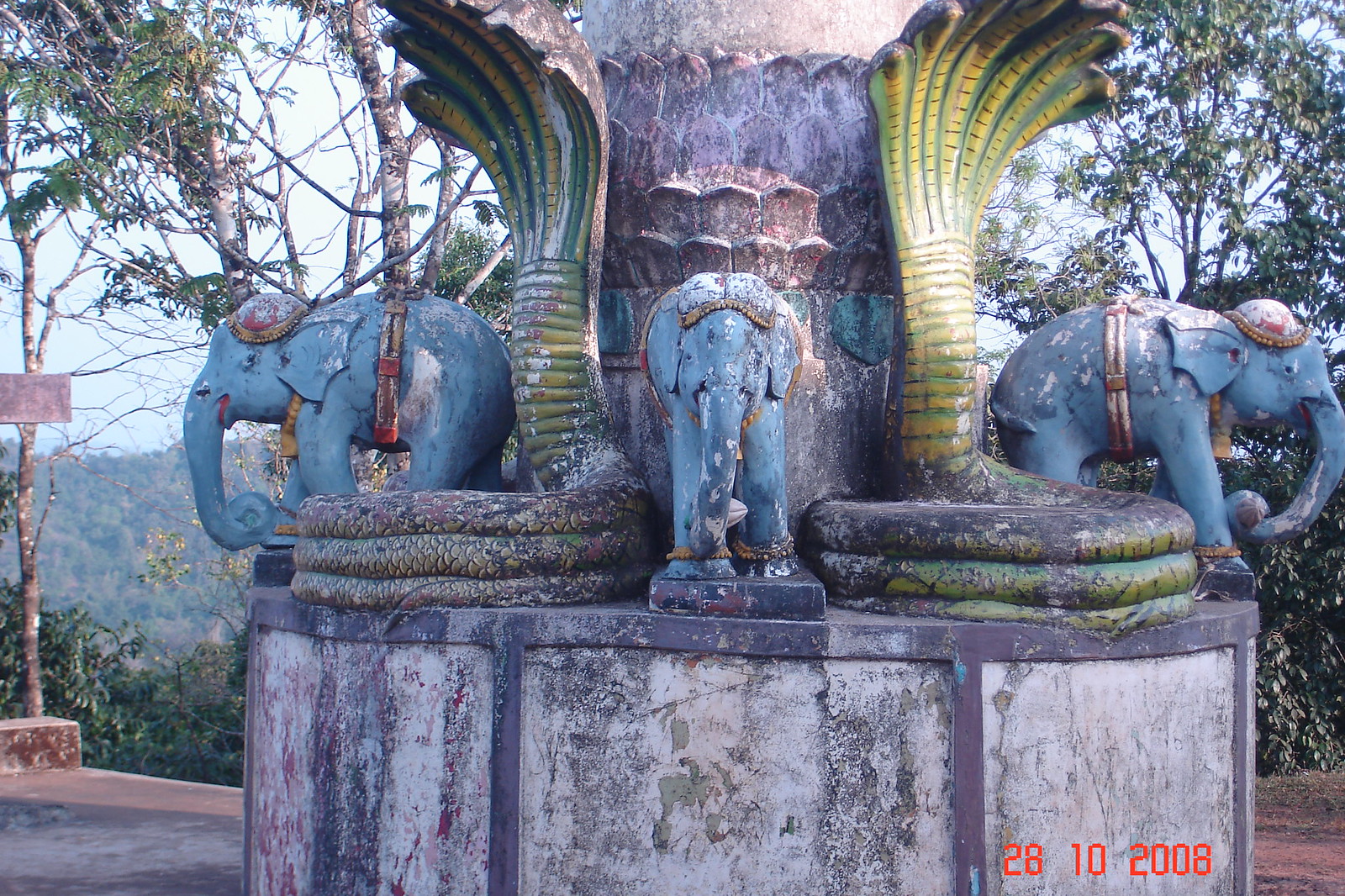This photograph, taken on 28-10-2008, captures a weather-beaten and somewhat dilapidated sculpture set against a backdrop of a blue sky with green, narrow trees. The structure, possibly an old water fountain, is situated on an elevated position overlooking a valley of mountains and vegetation. The base is circular and made of white stone with a chipped and moldy brown-to-gray border. The top of the structure features three statues of blue elephants adorned with red headdresses, positioned facing forward, left, and right. In between these elephant statues, there are two coiled snake-like figures, possibly cobras, depicted in green and yellow. These snake statues rise and fan out towards the top, although the top sections are cut off in the image. The base has sections of light purple and dark purple, with dark purple supports between the sections, and the entire structure is set on what appears to be a concrete ground with a red border.